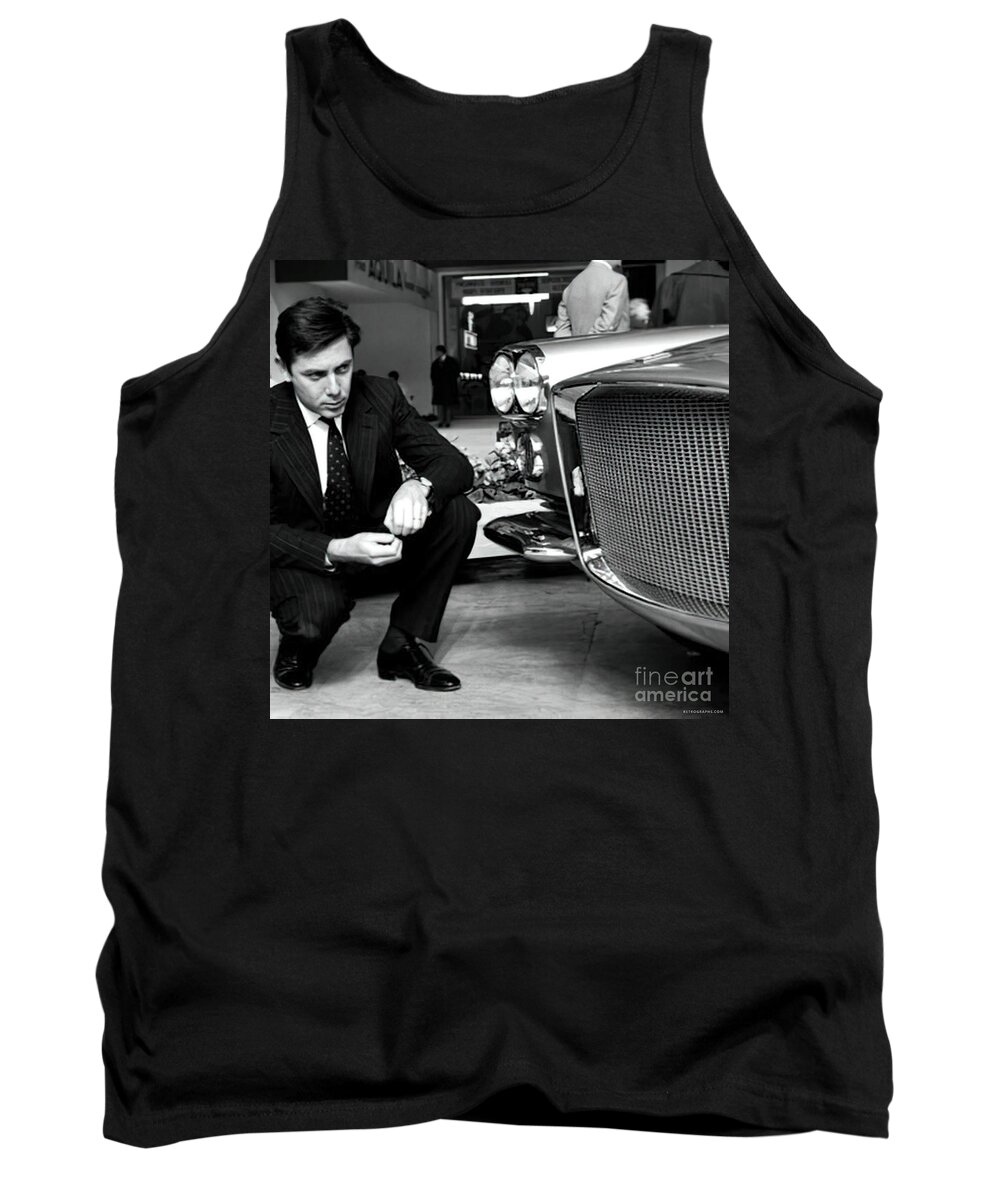This image depicts a black sleeveless muscle tank top featuring an intricate black and white print on the front. The printed image shows a man in a dark, possibly pinstriped suit with dark hair, black dress shoes, and a patterned tie, kneeling down and looking at the front grille and headlights of a luxury automobile positioned on the right side of the graphic. The bottom right corner of the image contains the text "Fine Art America." In the background, there are glimpses of another man’s back and shoulders, parts of a building possibly resembling a parking structure or deck, along with installed ceiling lights. Additionally, a few more figures can be seen in the distant background, standing around the scene.